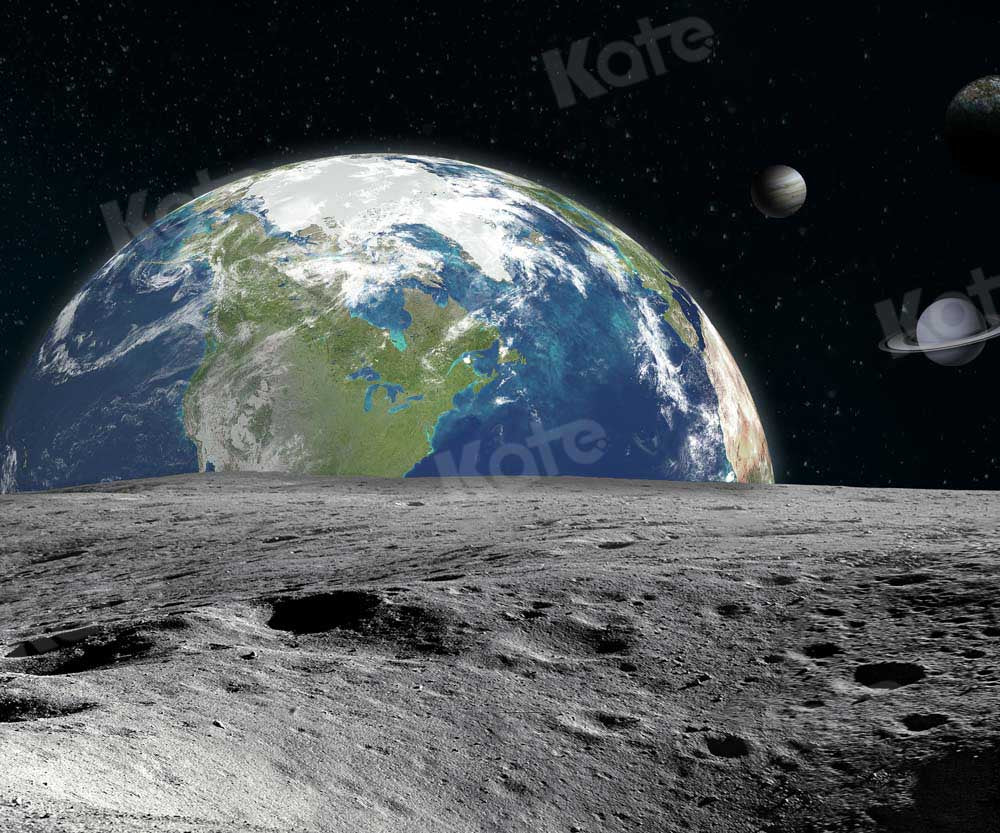In this image, we see a detailed and artistic representation of an outer space view. It presents Earth as seen from the moon, with North America prominently visible. The Earth appears unusually close to the moon, suggesting artistic license with the scale. The foreground depicts a rocky and pockmarked lunar surface, marked with craters and what appear to be footprints from astronauts. The background is a stark, black sky speckled with tiny white stars.

To the right of the image, there's a planet with a ring around it, closely resembling Saturn, and above it to the left, another planet without rings, likely Jupiter. Both planets are far closer to each other and to the moon than they would be in reality, adding to the surreal quality of the scene. The entire image is in black and white, enhancing the stark contrast and detail. A watermark reading "K-A-T-E" is superimposed across this celestial tableau. The celestial bodies and the artistic elements suggest that some of the planets may have been digitally placed into the scene, contributing to its dreamlike appearance.